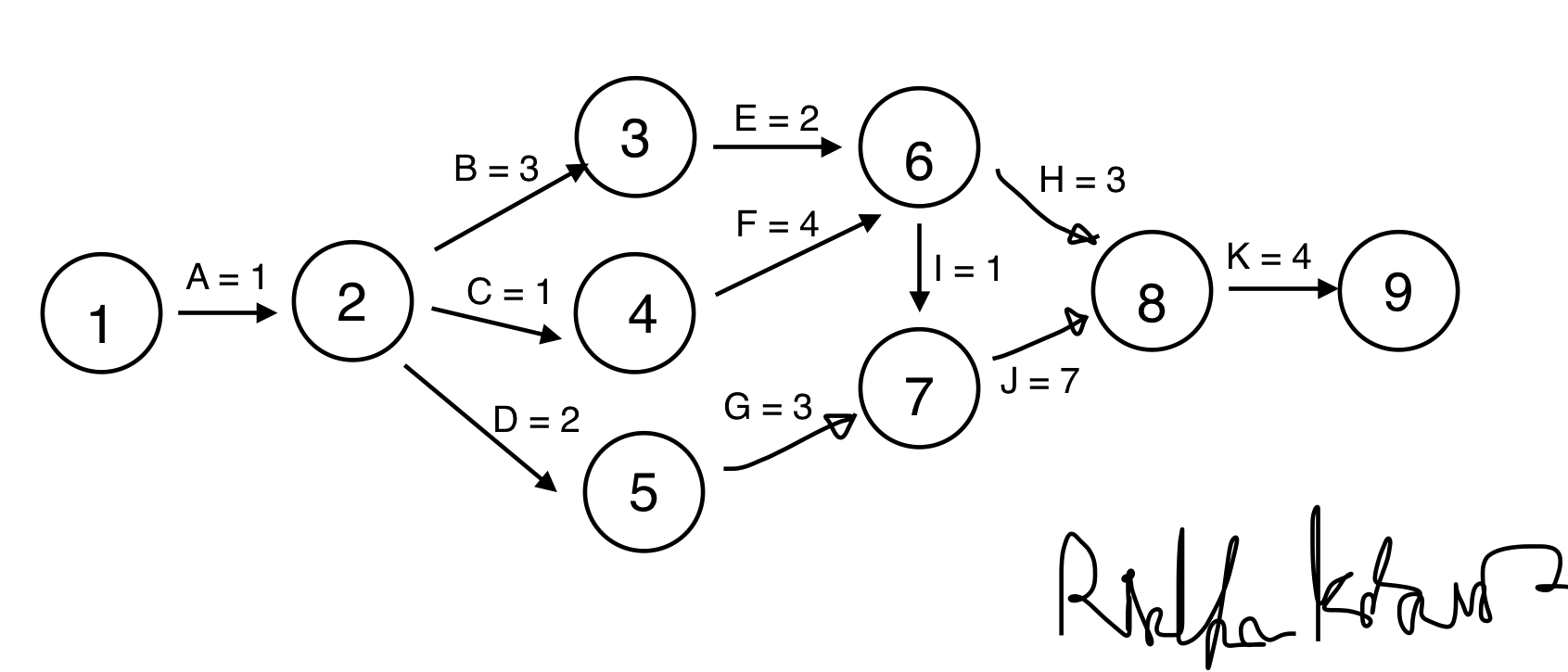A detailed, cleaned-up caption for the image might be:

"This image displays a structured math diagram, characterized by a series of circles and arrows connecting various numbers. The circles are sequentially numbered from 1 to 9. An arrow originates from the circle labeled '1' pointing to the circle labeled '2', which then connects to circle '3'. Additional arrows branch out from circle '2', leading to circles '4' and '5', continuing this pattern throughout the image. In the bottom right-hand corner of the diagram, a name is scribbled starting with an 'R' and a last name beginning with 'K', possibly 'Ralph K…'. The diagram includes a key where 'A = 1', 'B = 3', 'C = 1', and 'D = 2', applying these values across the entire picture."